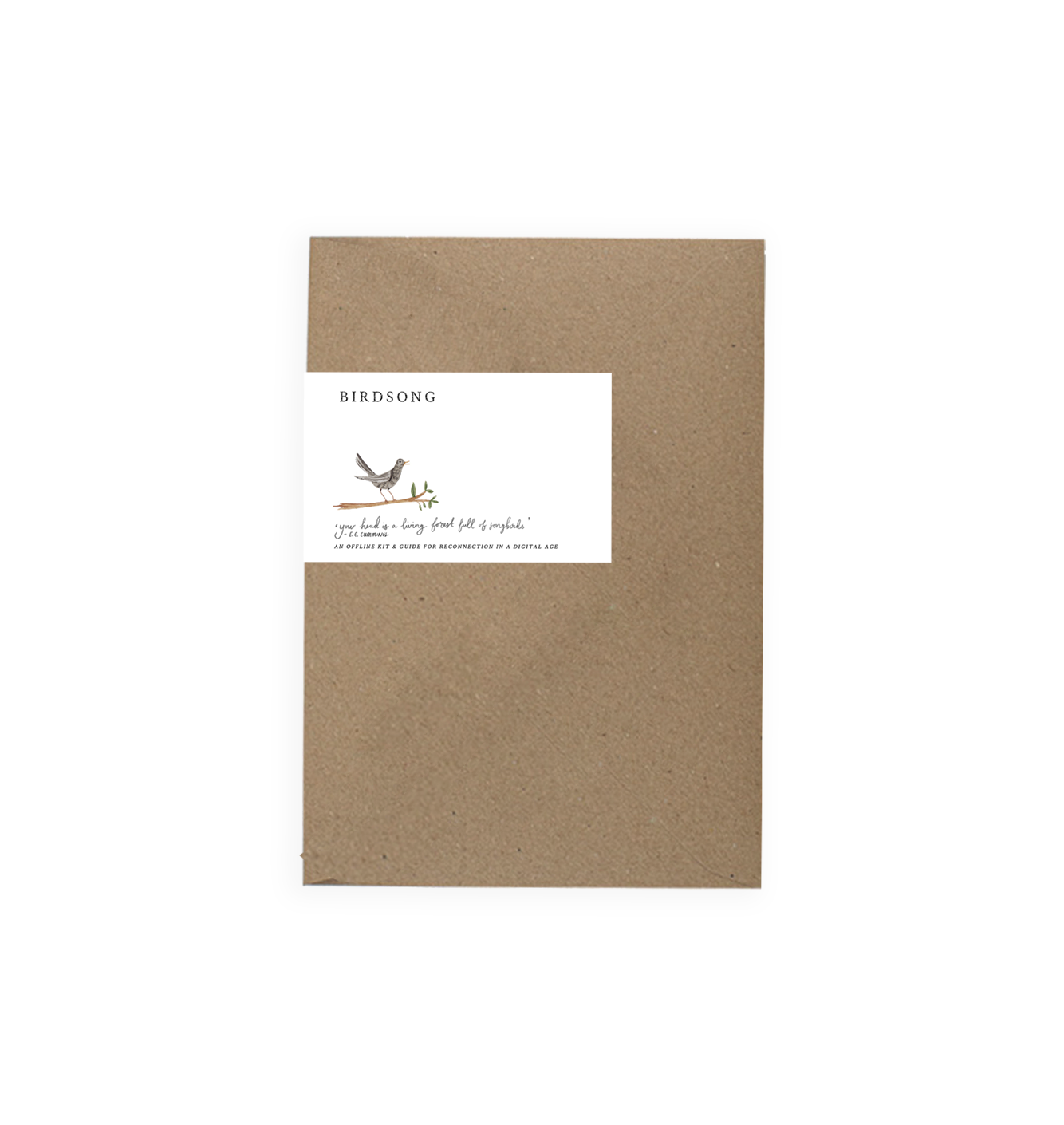The image depicts a meticulously detailed book cover or poster, featuring a central white triangle overlaying a brown background. Across the top of the white section, the word "Birdsong" is elegantly inscribed in black text. Below the title, a skillfully drawn bird with shades of purplish gray perches gracefully on a light brown branch, which is adorned with fresh green leaves. The bird is characterized by its long tail pointing upwards and wings that lay flat against its body, emphasizing its poised stance. The lower portion of the white triangle contains additional text, which despite being too small to read clearly, suggests phrases related to nature and reconnecting in the digital age. This piece, with its combination of artistic representation and textual elements, evokes an appreciation for nature and the simplicity of life. The setting of the image appears to be on a gray surface that could resemble a bulletin board or background, lending a natural, earthy ambiance to the overall composition.